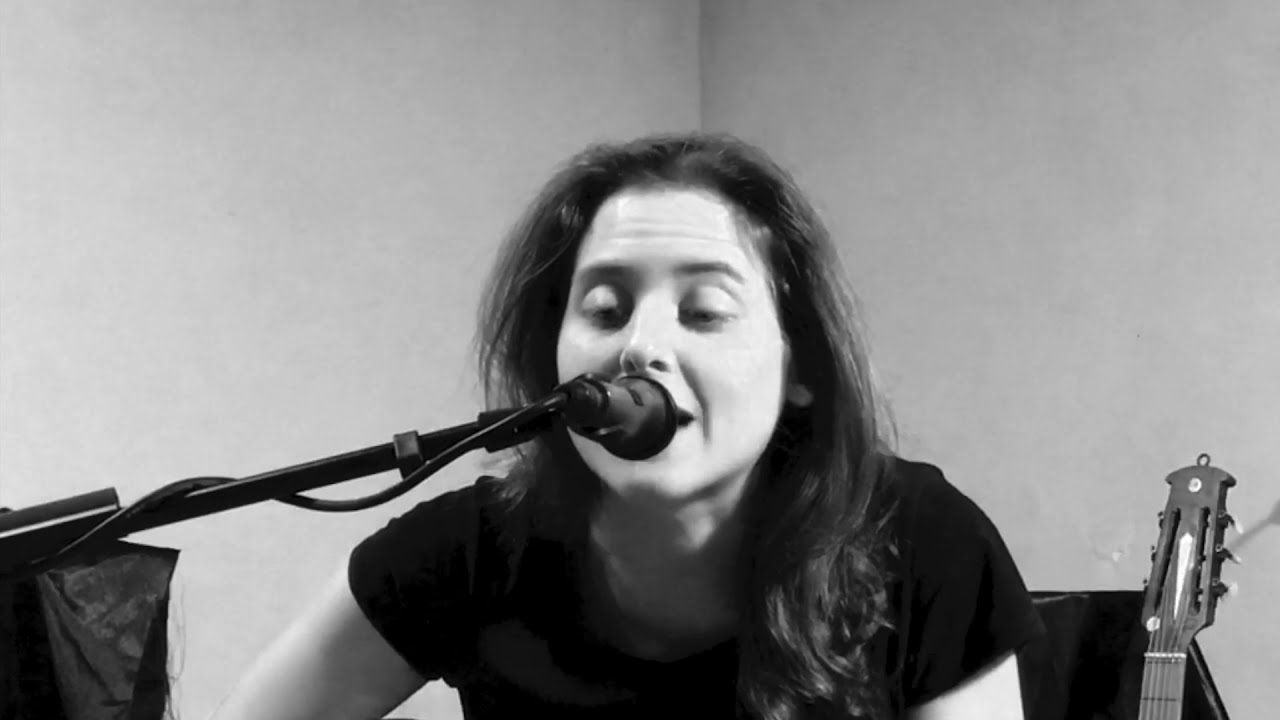In this horizontal rectangular black-and-white photograph, a young woman in her mid-20s is captured singing into a microphone. She is positioned in the corner of a room, with the crease mark between the two white or gray walls clearly visible in the background. The microphone, attached to a stand, extends from the lower left corner of the image towards the center, where the woman leans in, mouth open as she sings. Her longer dark brown or black hair falls past her shoulders, with slight curls at the ends. She wears a short-sleeve black t-shirt, and her brown eyebrows are noticeable above her open, downcast eyes. The top part of a guitar, including the headstock and tuning pegs, is visible in the lower right corner of the photo. Additionally, a piece of black fabric, possibly a bag or scarf, is seen in the lower left corner, adding to the minimalistic setting with bare walls.